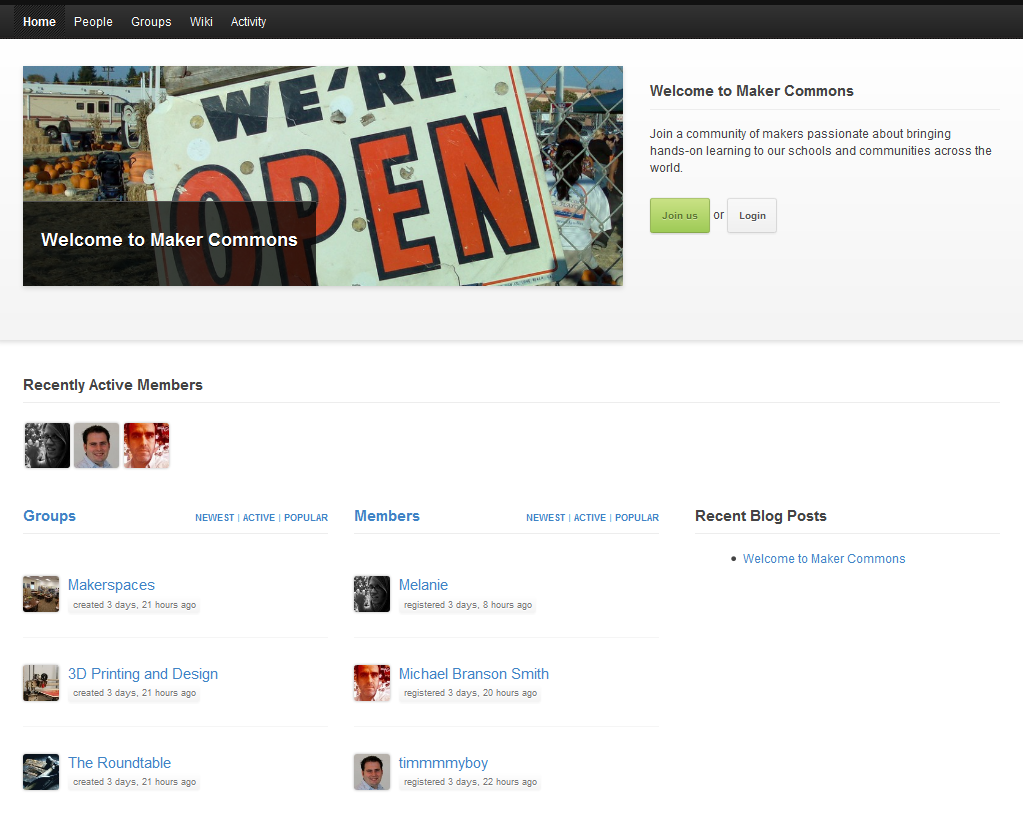This screenshot captures a web page from Maker Commons, a community platform for makers who are committed to integrating hands-on learning into schools and communities globally. 

### Header
At the very top, a thin black bar stretches horizontally across the page, featuring several menu options on the left: Home, People, Groups, Wiki, and Activity. The "Home" tab is currently selected.

### Main Section
Beneath the menu, a prominent gray box occupies the upper section of the page. On the right side of this box, there's a welcome message that reads: "Welcome to Maker Commons. Join a community of makers passionate about bringing hands-on learning to our schools and communities across the world." Below this message, there are two buttons: a green "Join Us" button and a gray "Log In" button.

To the left, there is a stock image—a long rectangular photo displaying a white sign that says "We're Open." The word "We're" is in black text, while "Open" is in large, orange capital letters outlined in black. The background of the image shows a pumpkin patch with people milling around, suggesting an outdoor fair or event. A dark gray overlay text box on the image reads "Welcome to Maker Commons" in white text.

### Bottom Section
The bottom half of the page features a white background with various sections. On the left, under the heading "Recently Active Members," three member profiles are listed. Below this, sections for "Groups" and "Members" include filters for "Newest," "Active," and "Popular." Another section titled "Recent Blog Posts" lists various posts, such as:
- "Maker Spaces," created 3 days and 21 hours ago.
- "3D Printing and Design," created 3 days and 21 hours ago.
- "The Roundtable," created 3 days and 21 hours ago.

### Member Activity
The "Members" section highlights recent registrations, featuring:
- Melanie, registered 3 days and 8 hours ago.
- Michael Branson-Smith, registered 3 days and 20 hours ago.

This detailed layout aims to create an engaging and welcoming environment for new and existing members of Maker Commons.